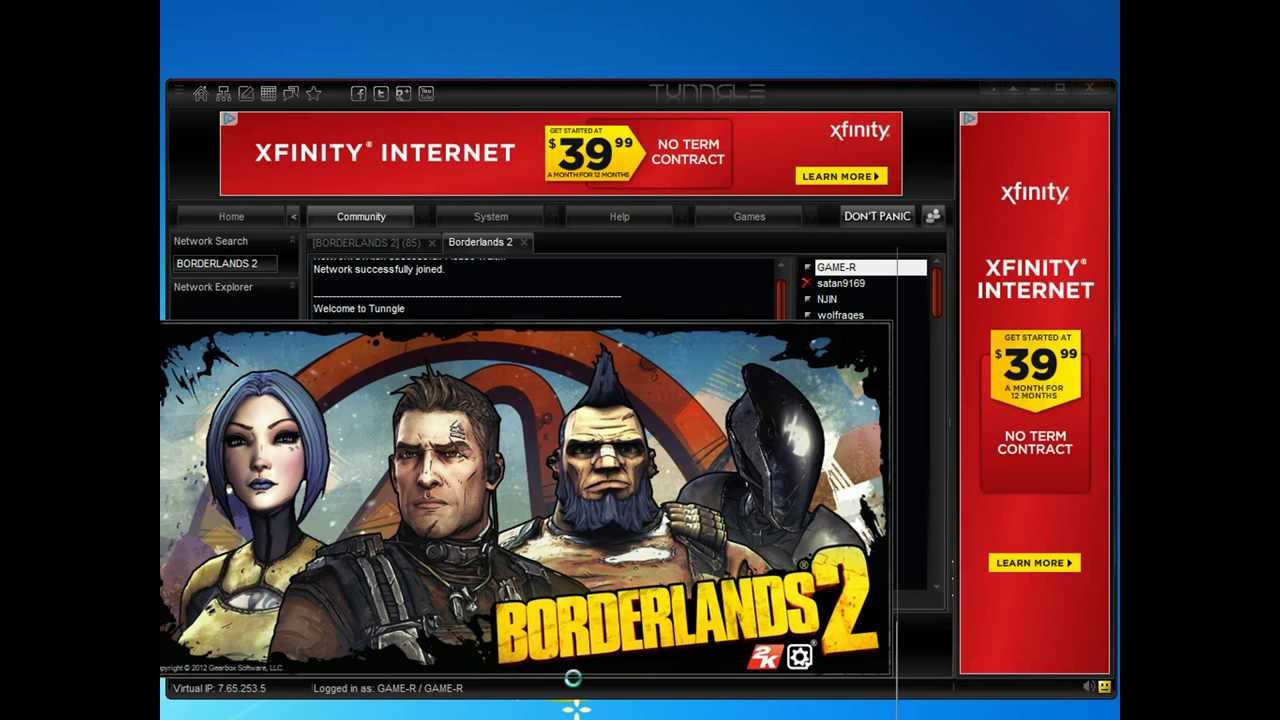This image showcases a website interface brimming with various interactive elements. Dominating the bottom of the screen is a prominent blue bar containing an array of white icons; there are seven assorted icons on the left, flanked by a gap, and then followed by four more white box-shaped icons. Centrally positioned within this bar, the word "Tungle" (spelled T-U-N-N-G-L-E) is prominently displayed in white text, flanked on the right by five additional, indistinct symbols.

Beneath this central navigation area, a striking red box stands out, featuring the words "Xfinity Internet" in white typeface. Adjacent to this, a yellow tag highlights the price "$39.99," and the phrase "No Term Contract" is clearly printed in white nearby.

Further down the page, a menu bar with various options spans horizontally from left to right, containing labels for "Home," "Community," "Explore," "Help," "Games," and an intriguingly titled section, "Don't Panic."

Anchoring the visual section of the webpage, a captivating image of a popular game is prominently displayed. This action-packed scene from "Borderlands 2" features four vividly detailed characters in the spotlight. On the far left stands a woman with striking short blue hair. In the immediate foreground, a rugged man clad in military-style armor stands prominently with his face exposed. To his right, a muscular character with a black mohawk and a beard exudes strength. Further right is a mysterious figure, fully covered in a sleek black suit with an obscured face. The iconic "Borderlands 2" title is emblazoned in bold yellow text in the bottom right-hand corner of the image, adding a dynamic touch to the overall composition.